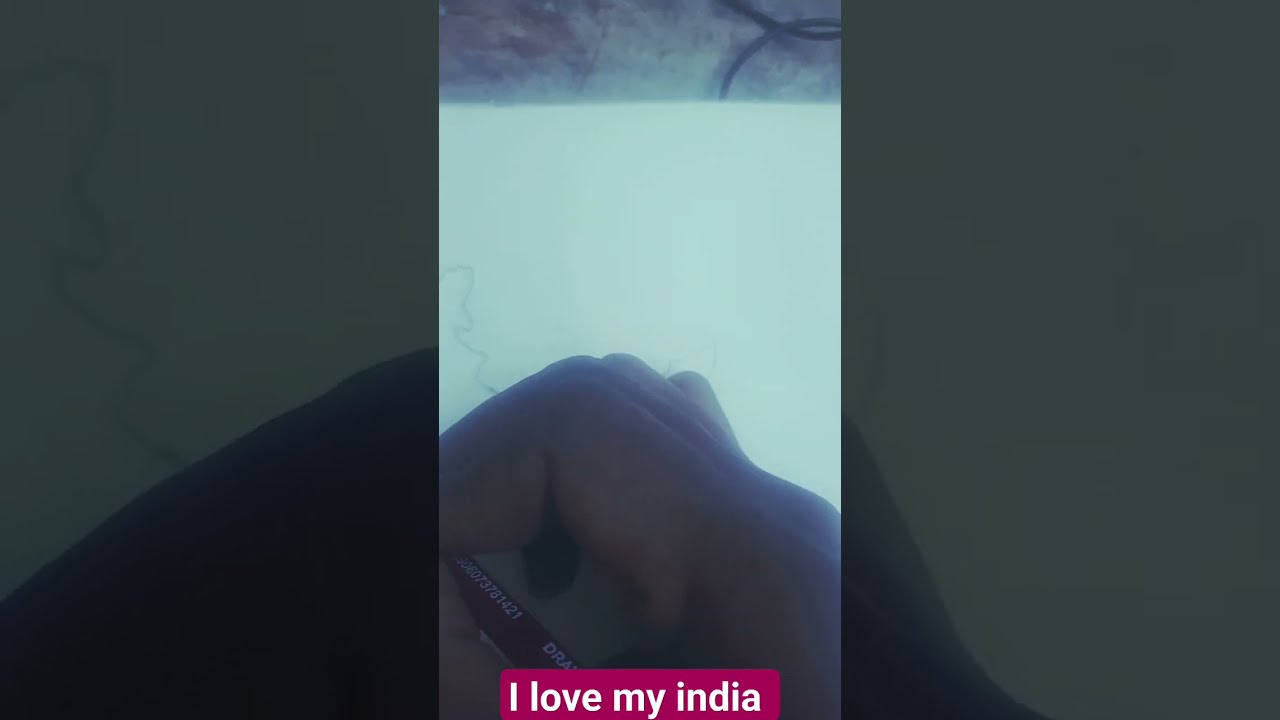A detailed close-up image shows the left side of a person's hand, where their fingers ascend, bend in the middle, and descend again. A black bracelet with white letters, displaying the characters "DRA," encircles the wrist, while the accompanying numbers remain too small to decipher. Below the hand, nestled in a maroon rectangle, white text reads "I love my India," with 'India' notably spelled using lowercase 'i's. The background features a hazy blue atmosphere, likely a snowy field with steam rising, and at the very top, distant trees transition from darker green on the left to lighter towards the center. A distinctive black swirl emerges on the right, curving up and out of the frame.